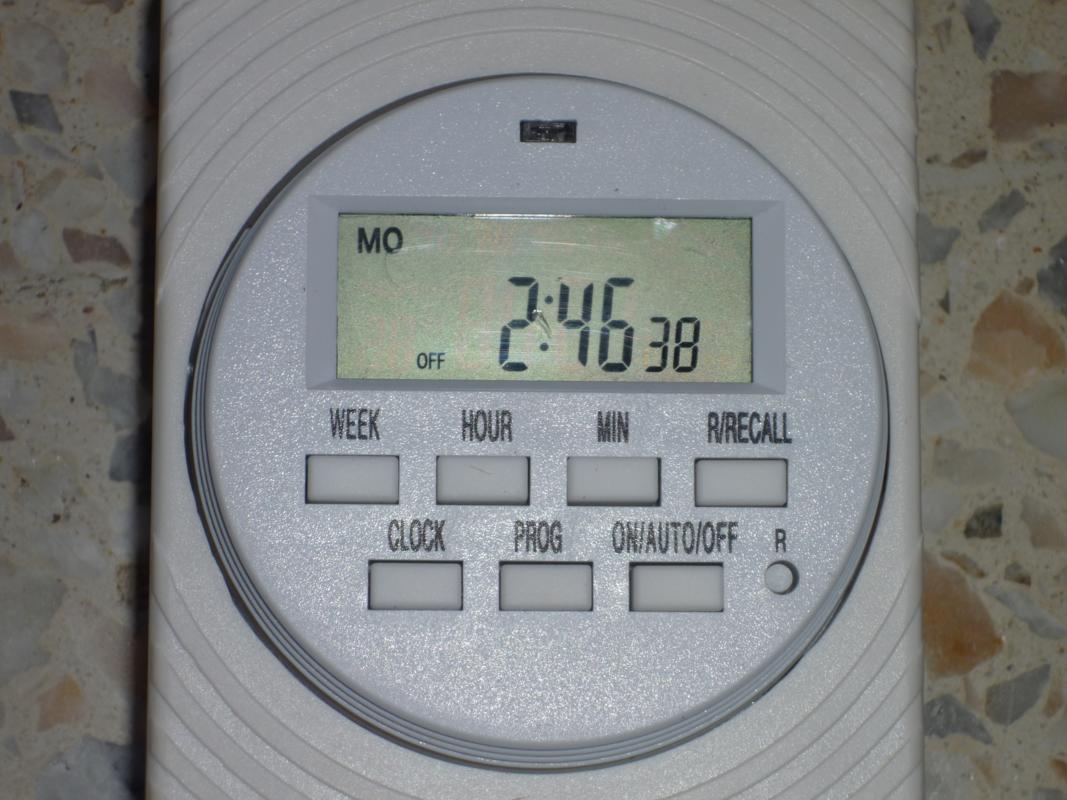This photograph features a programmable thermostat set against a cream-colored background adorned with small shapes in hues of brown, blue, gray, and peach. The thermostat itself is a clean, white rectangular device, prominently showcasing a central white circle bordered by a gray outline. Protruding subtly from the top and bottom of this circle are raised half circles, adding a tactile dimension to the design. 

At the apex of the central circle is a small, blocky rectangular indentation. Directly below it lies a recessed digital display, characterized by a distinct green-yellow hue. In the top left corner of the display, the characters "MO" are displayed in black uppercase letters. Towards the bottom left corner of the display, the word "off" can be seen in black, adjacent to large digital numbers reading "2:46", with a smaller "38" displayed beside them.

Beneath the digital display are four aligned rectangular buttons, each labeled respectively with "week", "hour", "min", and "r/recall". Below this row is a trio of horizontally arranged buttons, marked "clock", "PROG", and "on/auto/off". To the far right of these buttons, a small round button is labeled with an "R" above it, completing the intricate and functional layout of the thermostat.